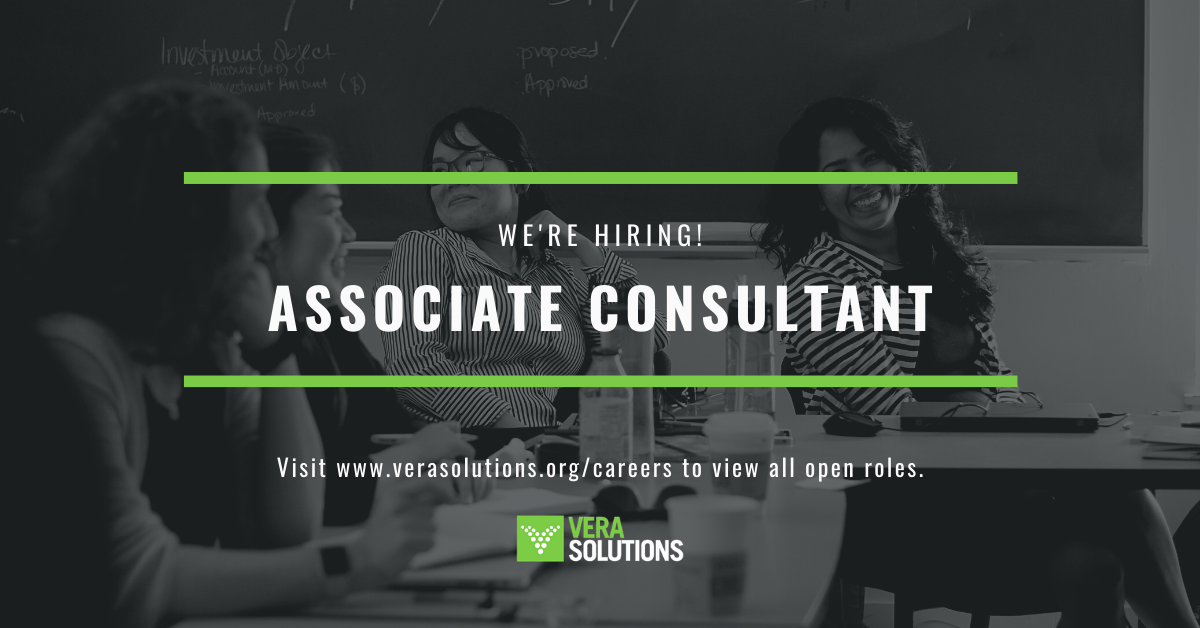A minimalistic webpage prominently features a black-and-white photograph as its background, depicting four women seated at a table, engaged in conversation and smiling. On the table, there are water bottles and at least one coffee cup visible. Overlaying the image are several elements: a horizontal green bar with the text "We're Hiring! Associate Consultant" in white, followed by another green bar stating "Visit www.VeraSolutions.org/careers to view all open roles." Beneath these bars is a green square containing white dots forming a 'V,' alongside the text "Vera" in green and "Solutions" in white. The overall design creates a professional and inviting visual, encouraging visitors to explore career opportunities with Vera Solutions.